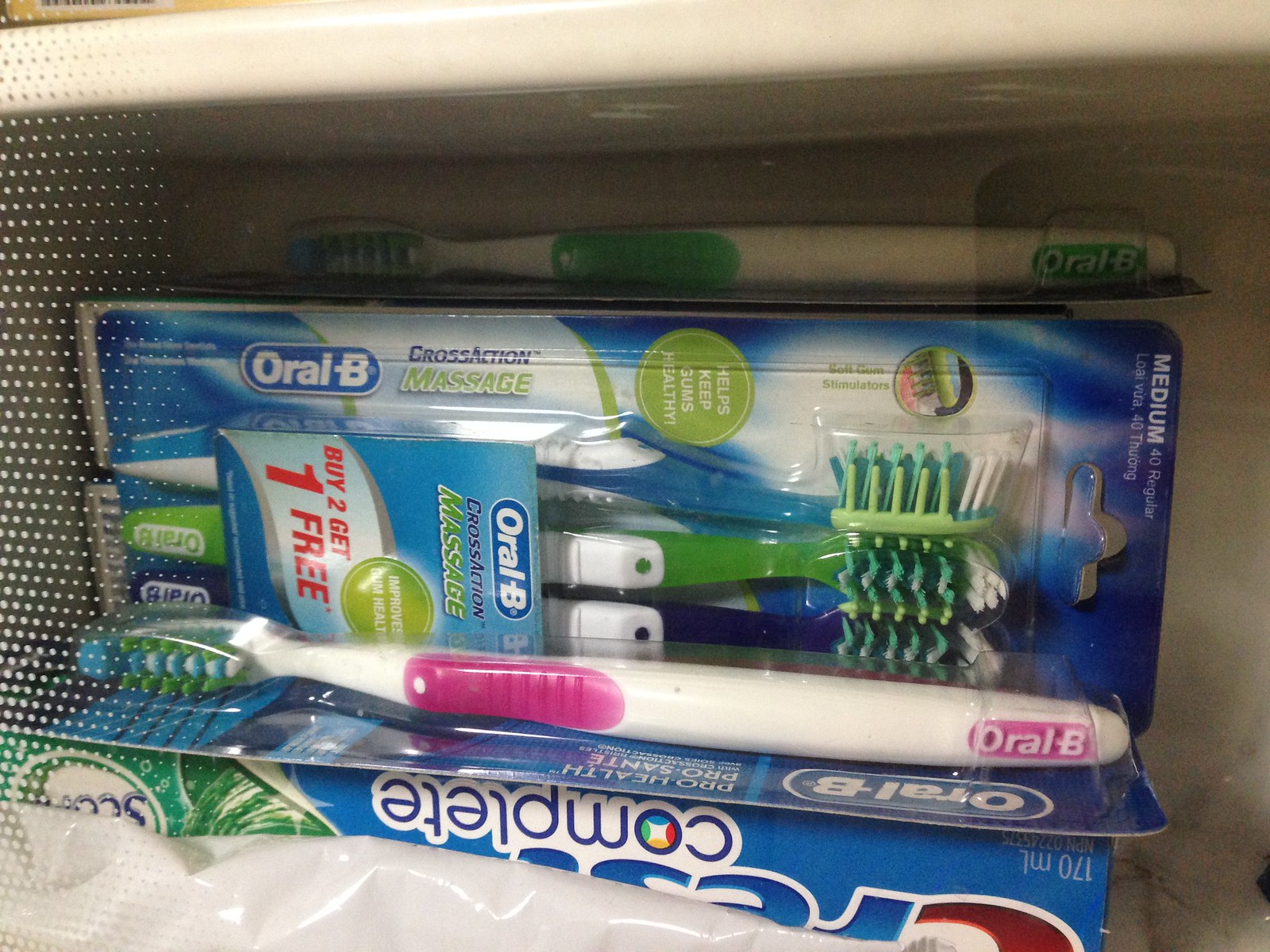Inside a beige-colored plastic container, there's an array of toothbrushes and a tube of toothpaste. At the bottom rests an Oral-B toothbrush featuring a green handle and white grip area. Nearby lies an unopened pack of Oral-B toothbrushes, showcasing a variety of colors: blue, green, and yellow handles with bristles in green, white, and blue. An additional pink and white toothbrush remains sealed in its packaging. The toothbrushes are stacked on top of a tube of Crest Complete toothpaste, which prominently displays a large red 'C' and blue lettering spelling out 'Crest' with the word 'Complete' below. The label also includes 'SCOPE' within a green bottle illustration, accompanied by blue letters. Overall, the neatly organized items seem almost suspended, as if contained in a display case.